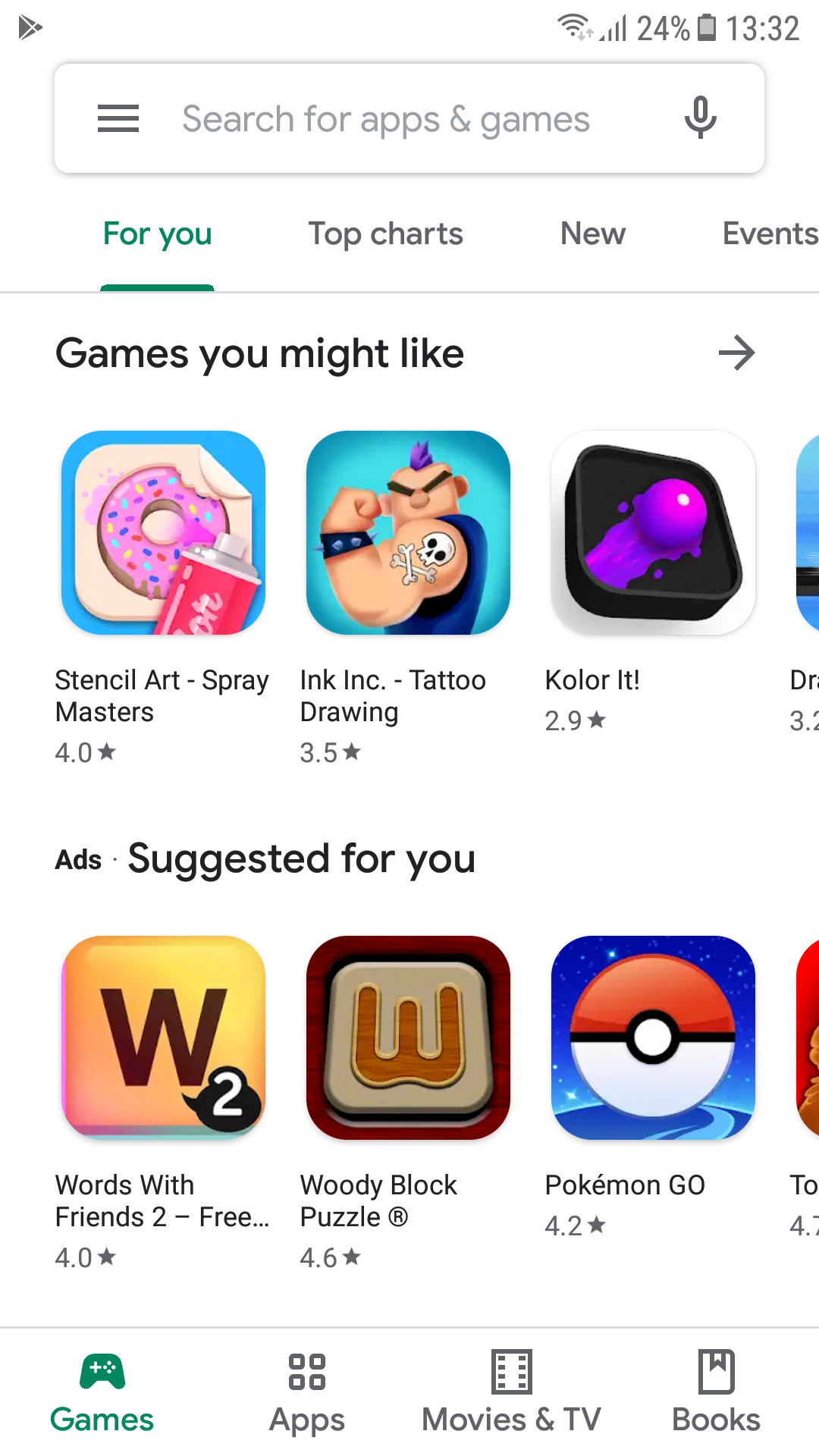The image depicts a screenshot of the Google Play Store interface. In the top-left corner, the gray Google Play Store symbol is visible. Next to it on the right, there is a Wi-Fi signal icon with arrows pointing up and down, indicating network activity. Further to the right, a full data service signal is represented with five out of five bars. Adjacent to this, the battery icon shows a 24% charge, and the current time displayed is 13:32.

Below the status bar, there is a rounded rectangular search bar with the placeholder text “Search for games and apps” in light gray. To the right of the search bar, a dark gray microphone icon is present, and to the left, three dark gray horizontal lines represent a menu.

Underneath the search bar, there are menu options such as "For You," "Top Charts," and "New Events." The "For You" section is highlighted in dark green, with a thick dark green line beneath it. The section header reads “Games you might like” in bold black letters with an arrow pointing right.

In the list of suggested games, the first icon is for "Stencil Art Spray Masters," displaying an image of a spray-painted doughnut on a piece of paper that is folding at the upper right-hand corner. The next game, "Ink Inc. - Tattoo Drawing," shows a cartoon figure with a skull tattoo on their bicep and a Mohawk. Another app, "Color It," features a slanted perspective with a prominent purple paint ball. It shows a rating of 2.9 stars.

At the bottom of the section, the text "Suggested for you" appears with "Ads" in small, bold black letters on the left. Below this, app icons for "Words with Friends," "Woody Block," and "Pokemon Go" are displayed.

The bottom navigation bar features icons for different categories: "Games," "Apps," "Movies & TV," and "Books."